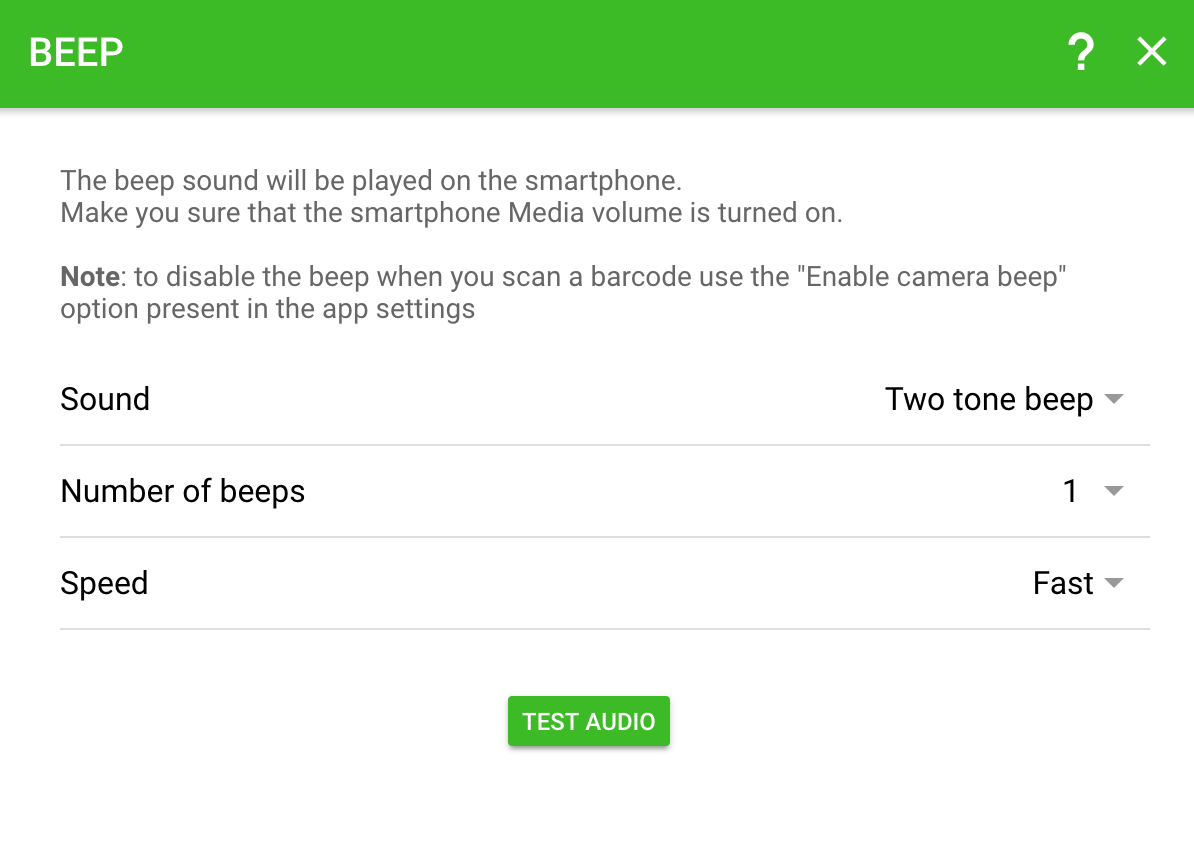The screenshot displays an interface from a mobile application on a standard phone or tablet. At the top of the screen is a thick green header with the text "BEEP" in all capital letters. In the far right corner of this header, there are two icons: a question mark and an 'X'.

Further down, towards the bottom, there's a green rectangle in the same color as the top header, containing white text that reads "Test Audio". Below this, in a standard font, the following message is displayed: "The beep sound will be played on the smartphone. Make sure that the smartphone media volume is turned on." This message is repeated, but with the grammatical error "Make you sure."

A bold note then states: "To disable the beep when you scan a barcode, use the 'Enable Camera Beep' option present in the app settings."

A larger section of text reads "Sound:", and next to it, "Two Tone Beep" has been selected from a dropdown menu. Beneath it, the "Number of Beeps" is set to one, and the "Speed" is configured as "Fast."